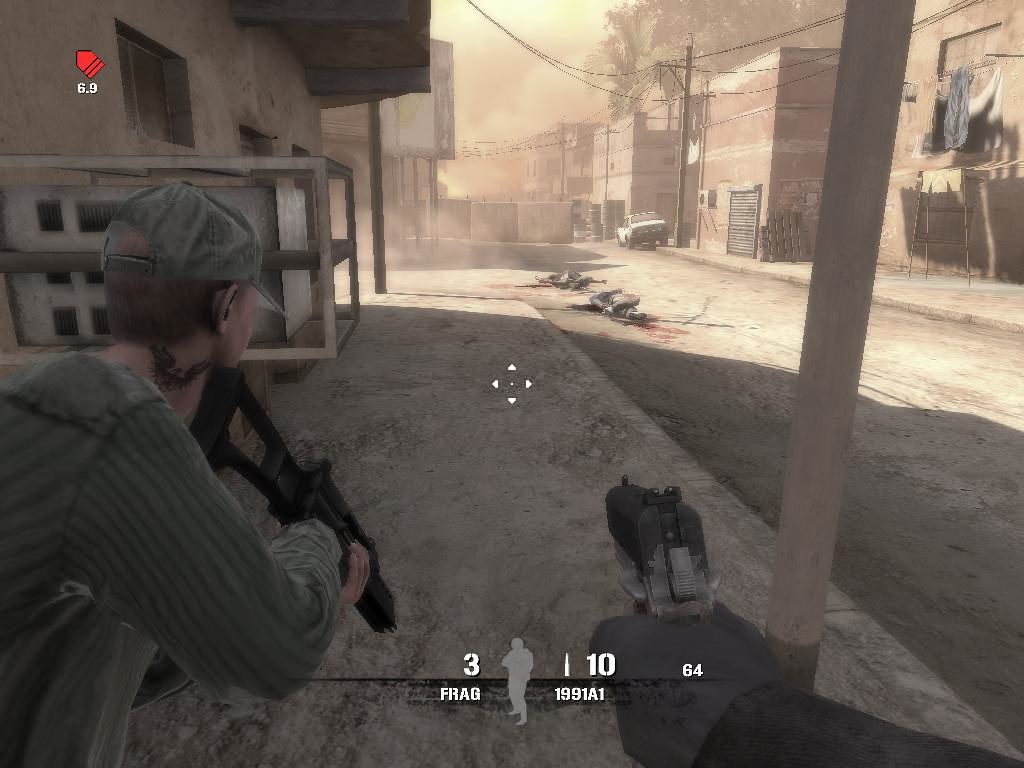This screenshot from a first-person shooter video game captures a tense urban scene. The primary player's view, shown from behind a dark hand gripping an automatic pistol with a black top and light gray bottom, emphasizes a white, cross-shaped crosshair with a central dot aimed forward. In the HUD, "3 frag" and "10" can be seen to the left, alongside "1991 A1" indicating the pistol's ammo, with a total of 64 bullets. To the left of the player, a character with short brown hair, an eagle tattoo on the neck, and attire consisting of a long-sleeved green shirt and green cap, wields a black rifle with a holed-out stock. This character stands against a tan building featuring a wooden-framed AC unit, casting shadows on the gray sidewalk alongside the dirt road strewn with bloodied bodies, under a yellow-orange sky. The background reveals a mix of red and tan buildings, telephone poles, clotheslines, and an old car, all shrouded in a sandstorm-like haze.